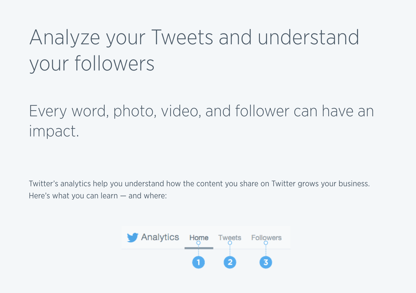A detailed Twitter analytics interface is shown. The design features a gray, horizontal rectangular box. At the top, bold letters proclaim, "Analyze your tweets and understand your followers." Below that, smaller text states, "Every word, photo, video, and follower can have an impact." Even smaller text explains, "Twitter's analytics help you understand how the content you share on Twitter grows your business. Here's what you can learn and where."

A blue Twitter bird logo appears next, accompanied by the word "Analytics." Below this, the word "Home" is underlined, indicating the current section. Underneath "Home," there is a vertical sequence starting with "1. Tweets," followed by "2. Followers," and finally "3. More." Each number is contained within a blue circle, suggesting clickable tabs for further exploration.